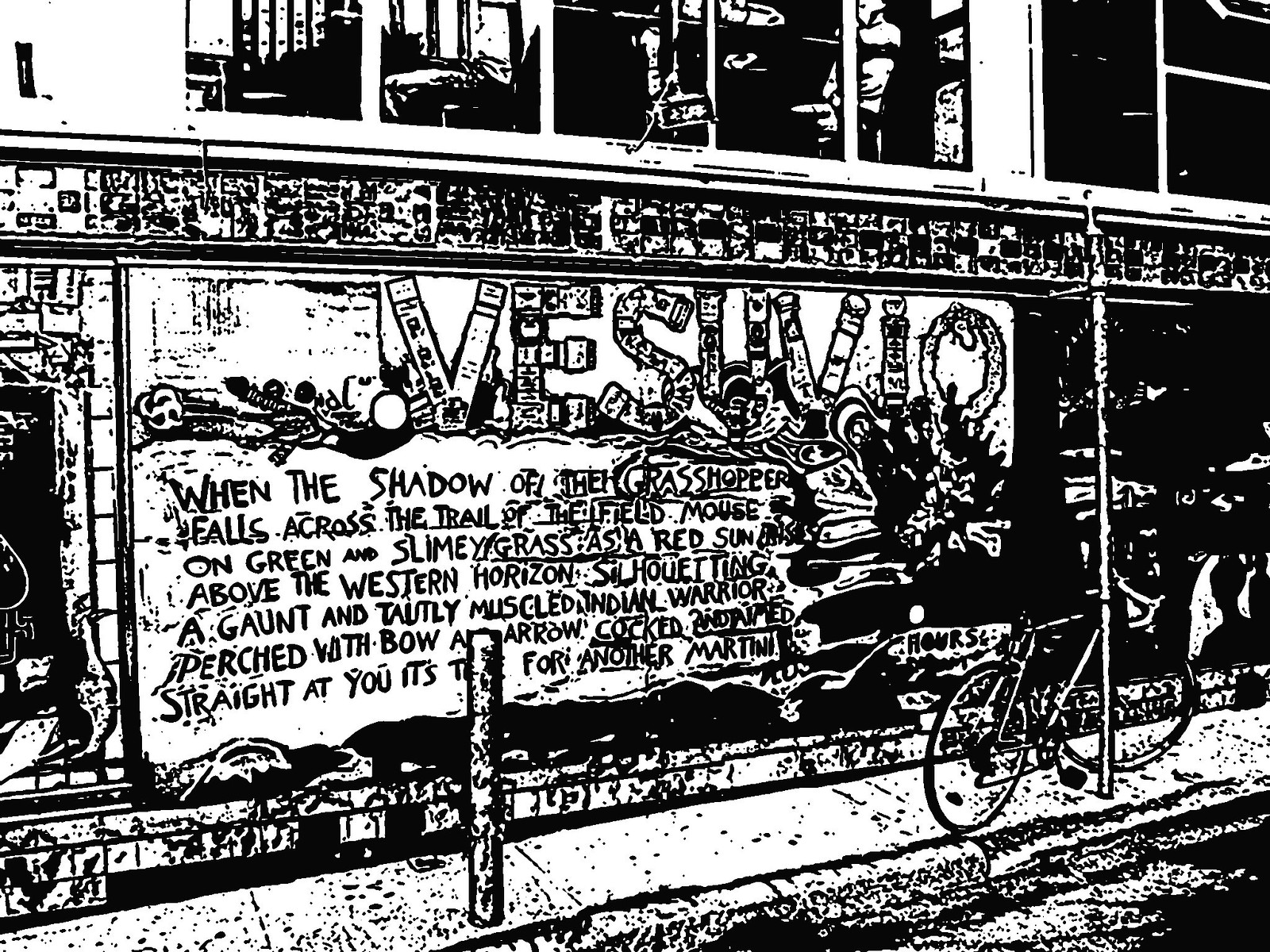The image is a detailed black-and-white graphic reminiscent of a comic strip or vintage newspaper advertisement. It features a busy street scene centered on a sidewalk and a storefront adorned with a mural that reads "Vesuvio." Below the name is a partially legible saying: "When the shadow of the grasshoppers falls across the trail, the field..." The right portion of the saying is cut off. The storefront appears to promote an establishment, perhaps a pub or bar named Vesuvio. Attached to a signpost on the sidewalk is a 10-speed bicycle, standing unattended. Another smaller post is nearby. Above the mural, the building extends at least two stories high, with darkened windows that possibly show a person seated inside, giving the impression of an apartment or office building. The graphic has intricate shadowing and shading, which adds depth and a slightly cluttered feel to the scene. Overall, it captures the essence of a bustling city corner with a nostalgic, old-time ambiance.